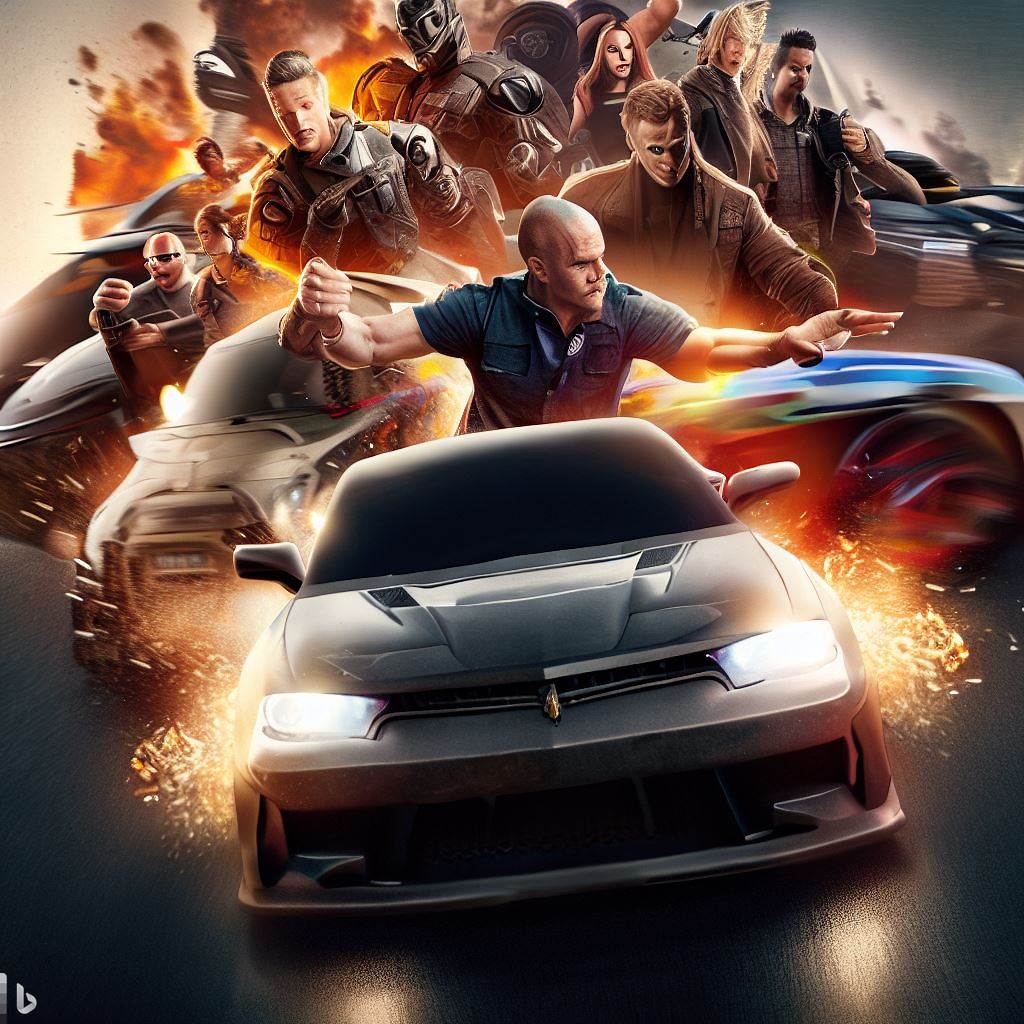This image appears to be an AI rendering of a high-octane action movie poster, with a clear nod towards the Fast and Furious franchise. At the center is a black sports car with dynamic sparks or fire flying off its wheels, heading directly towards the viewer with headlights blazing. The foreground displays this car in sharp relief, while behind it, two other cars are crashing in a chaotic and unnatural position, with one facing sideways and the other deformed in both the body and hood.

In the background stands a man, appearing to be a police officer or military figure, with grotesquely stretched arms and hands, likely a byproduct of graphical software artifacts. His bald head and nondescript face dominate the upper central part of the image. Surrounding him are incomplete and deformed renderings of various humans, hinting at men in military garb or riot gear. Some figures are wearing sunglasses, others are masked, with a mix of both genders, though details remain blurred and indistinct.

The overall composition, with its surreal and distorted elements, highlights the artificial nature of the image and the imperfections common in AI-generated art. The background silhouettes of more cars and people add to the chaotic, action-packed atmosphere typical of movie posters, emphasizing speed, conflict, and a high-stakes narrative.